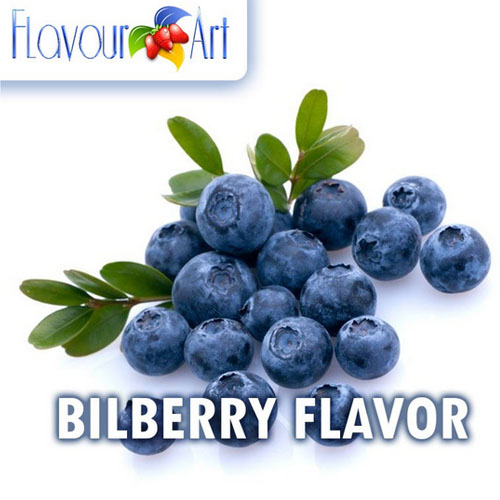The image features the text "Flavor Art" prominently displayed in the top left corner, though it should correctly read "FLA-VOUR." Below this text is the logo, which comprises three red berries, a yellow element beneath them, and a blue and green leaf intertwined in the word art. 

Dominating the image is an illustration of a handful of bilberries (distinctly labeled as "BILBERRY FLAVOUR" in white lettering), not to be mistaken for blueberries. There are about a dozen blue bilberries, each resembling a small paddle shape as if taken from an artist's palette. Among these bilberries, one particularly large bilberry stands out towards the left, positioned on top of another berry. This detailed depiction showcases bilberries adorned with small green leaves, adding a fresh and natural touch to the composition.